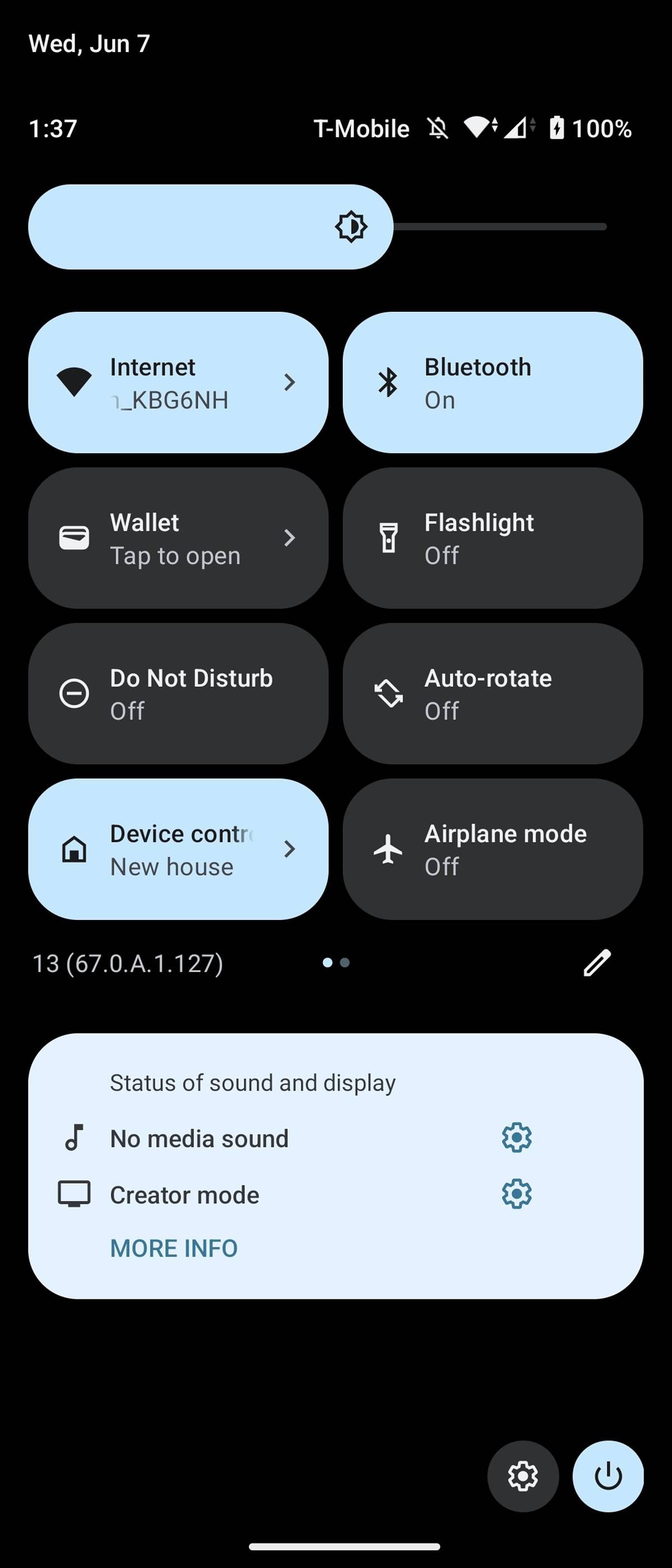This vertical image appears to be a screenshot taken from a smartphone. The background is a solid black, devoid of any texture or dimension, providing a flat visual effect. 

At the top left in white text, the date reads "Wed, Jun 7." Directly below this, the time is displayed as "1:37." On the top right, the text shows "T-Mobile" along with icons for notifications (a bell with a line through it), location services, and battery life at 100%.

A blue cylindrical bar is present below these details, featuring settings and account icons. Below this bar, the screen reads "Internet" accompanied by a triangle icon and a series of letters and numbers representing the Wi-Fi network. To the right, a Bluetooth icon indicates that Bluetooth is on.

Further down, within gray boxes, are additional system statuses: "Wallet" with a tap-to-open icon, "Do Not Disturb" which is off, "Flashlight" also off, "Auto Rotate" off, and "Device Control" for a smart home system, represented by a blue house icon. "Airplane Mode" is shown with its respective icon and is off.

Beneath these, it displays "13" followed by a number and letter in parentheses, likely relating to the status of sound or display settings. There's no media sound or creator mode active, and the bottom right corner of the screen shows icons for the power button and settings menu.